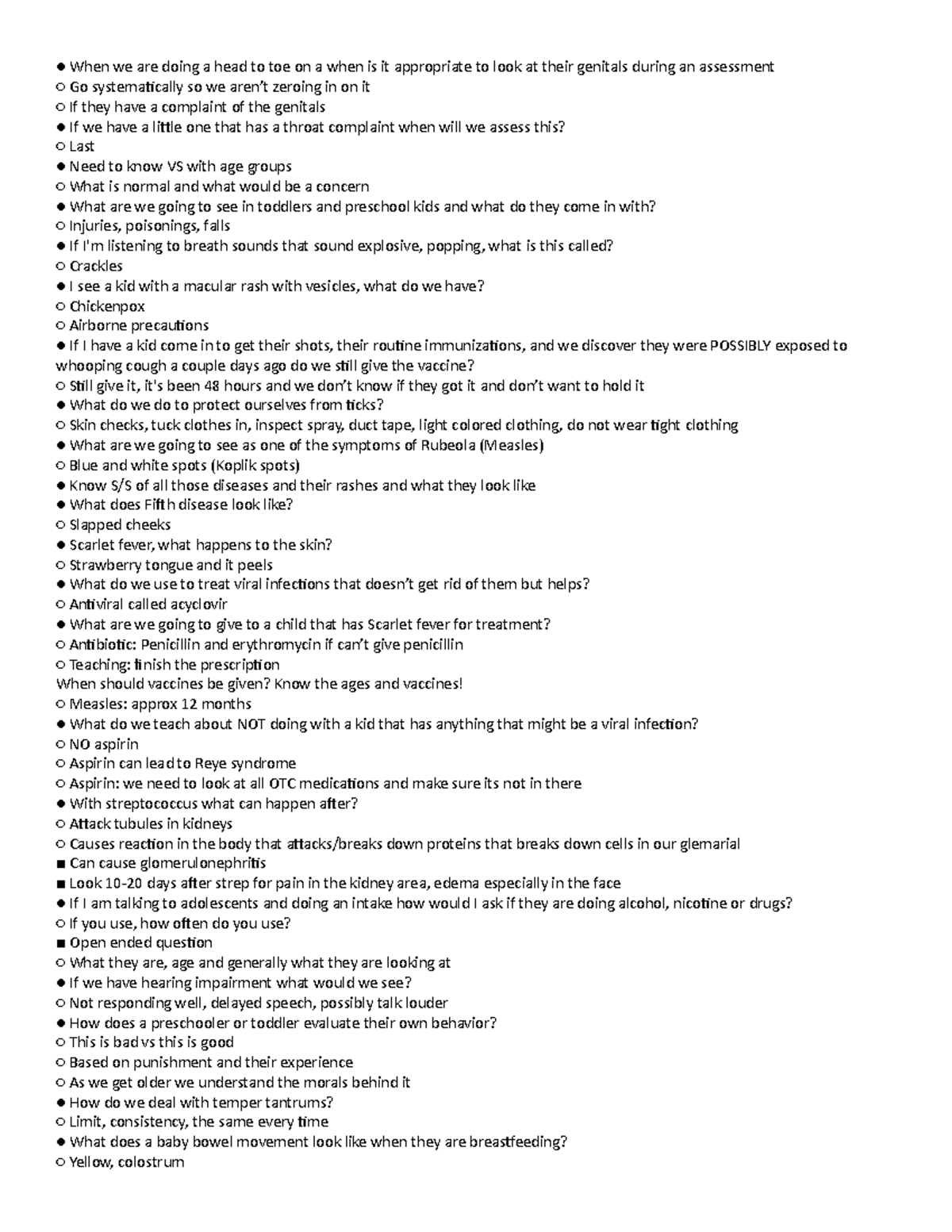The image captures a complex medical conversation or lecture, depicted through a detailed and systematic enumeration of various health assessments, symptoms, and treatments. In the scene, there are black dots, white dots, and black squares organized around the participants, possibly representing different medical conditions and protocols.

The dialogue indicates:
- The appropriate process for conducting a head-to-toe assessment, including when to examine a patient's genitals.
- Differences in examining patients based on age and specific complaints, such as genitals for specific issues, throat complaints for children, and the systematic assessment of symptoms.
- Recognition of various respiratory sounds like "crackles" and the identification of skin conditions such as macular rashes with vesicles indicating chickenpox, requiring airborne precautions.
- Vaccine protocols, including administering vaccines despite potential exposure to diseases like whooping cough.
- Measures to protect against ticks, including skin checks, tucking clothes, and using duct tape.
- Identifying symptoms of rubeola measles (blue and white spots, known as Koplik spots), fifth disease (slapped cheeks), and scarlet fever (strawberry tongue, peeling skin).
- Treating viral infections with antivirals like acyclovir and administering antibiotics like penicillin or erythromycin for conditions like scarlet fever.
- Teaching points on finishing antibiotic prescriptions and the appropriate ages for vaccines, such as measles at around 12 months.
- The dangers of providing aspirin to children with viral infections due to the risk of Reye's syndrome.
- Recognizing and managing post-streptococcal complications, including signs of glomerulonephritis like kidney pain and facial edema.
- Approaching sensitive topics with adolescents about substance use through open-ended questions.
- Identifying and managing hearing impairments and the differences in behavior evaluation between toddlers, preschoolers, and older children.
- Strategies for managing temper tantrums with consistent limits and understanding the characteristics of bowel movements in breastfed babies.

The image underscores a multifaceted and nuanced approach to pediatric assessment and care, involving thorough symptom recognition, appropriate testing and treatments, and careful consideration of developmental stages and patient education.